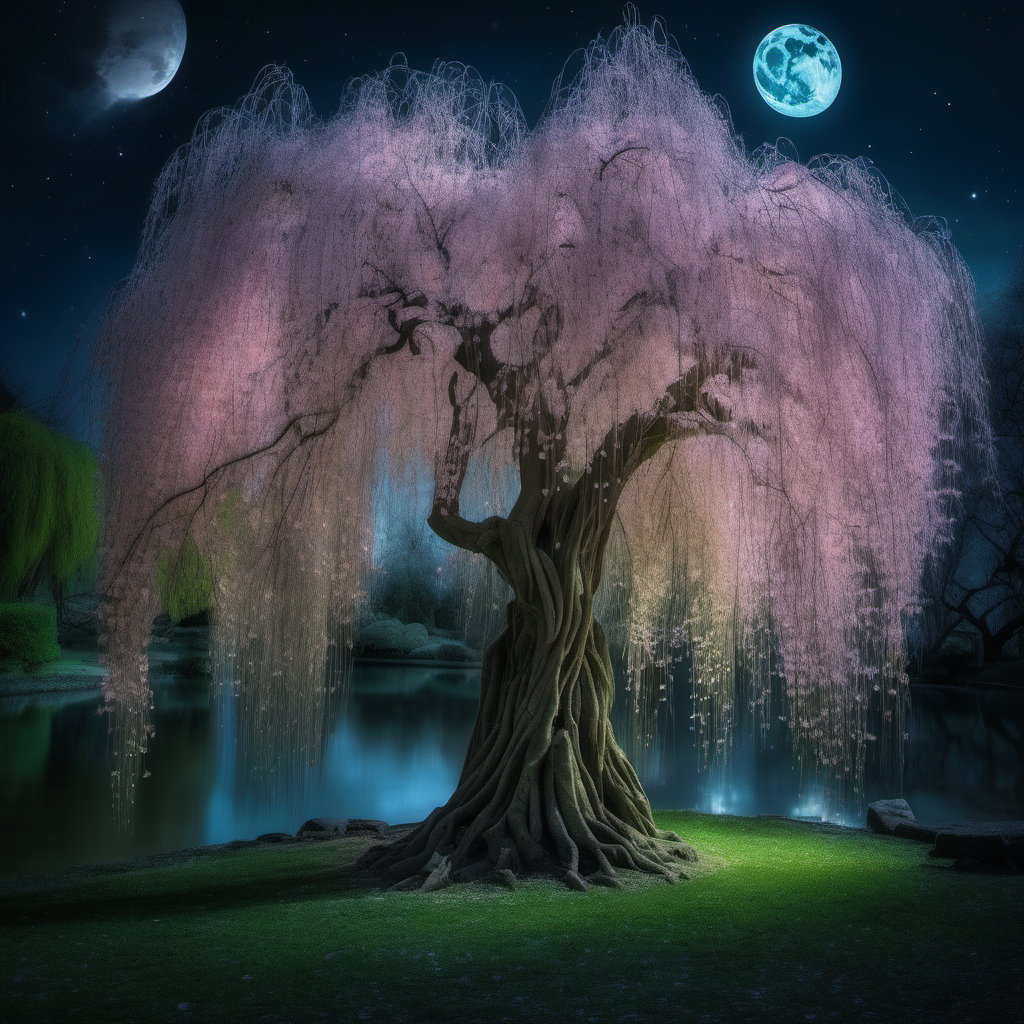In this enchanting fantasy scene, a somber night sky is dotted with sparkling stars, adding a touch of magic to the atmosphere. A luminous moon with intricate dark shapes casts a mystical glow, while another planet looms mysteriously on the left side of the horizon. Below, a lush expanse of vibrant green grass surrounds a serene little lake, creating a stark yet beautiful contrast to the celestial backdrop. Dominating the landscape is a large, eerie tree with gnarled roots that appear to climb up its twisted trunk. Cascading from its branches are ethereal, light purple leaves that hang like delicate strands of hair, lending the tree an otherworldly appearance. The scene as a whole is a mesmerizing blend of the eerie and the beautiful, capturing the imagination with its surreal elements.